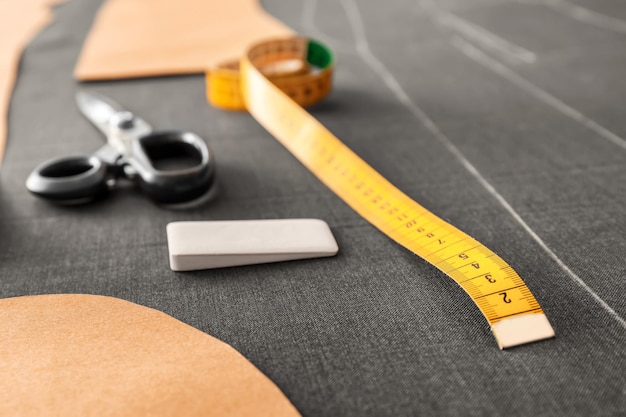This is a close-up, stylized photograph capturing a seamstress or tailor's essential tools laid out with meticulous detail. Dominating the scene is a flexible yellow measuring tape, curling towards the blurred background, purposefully placed on a piece of gray fabric. The measuring tape starts from two inches and extends into the distance, becoming fuzzy out of focus. Prominently displayed on the left are a pair of scissors with a black handle and silver blades, their metallic finish gleaming. Central to the composition is a white, wedge-shaped marking chalk, suggesting recent use for drawing stencil or chalk lines on the fabric. Surrounding these primary tools are pieces of tan-colored fabric, possibly leather, which lay cut and scattered atop the gray fabric, adding a tactile variety. The foreground is in sharp focus, highlighting the practical and artistic aspects of sewing, whereas the background blurs softly, hinting at an ongoing creative process.